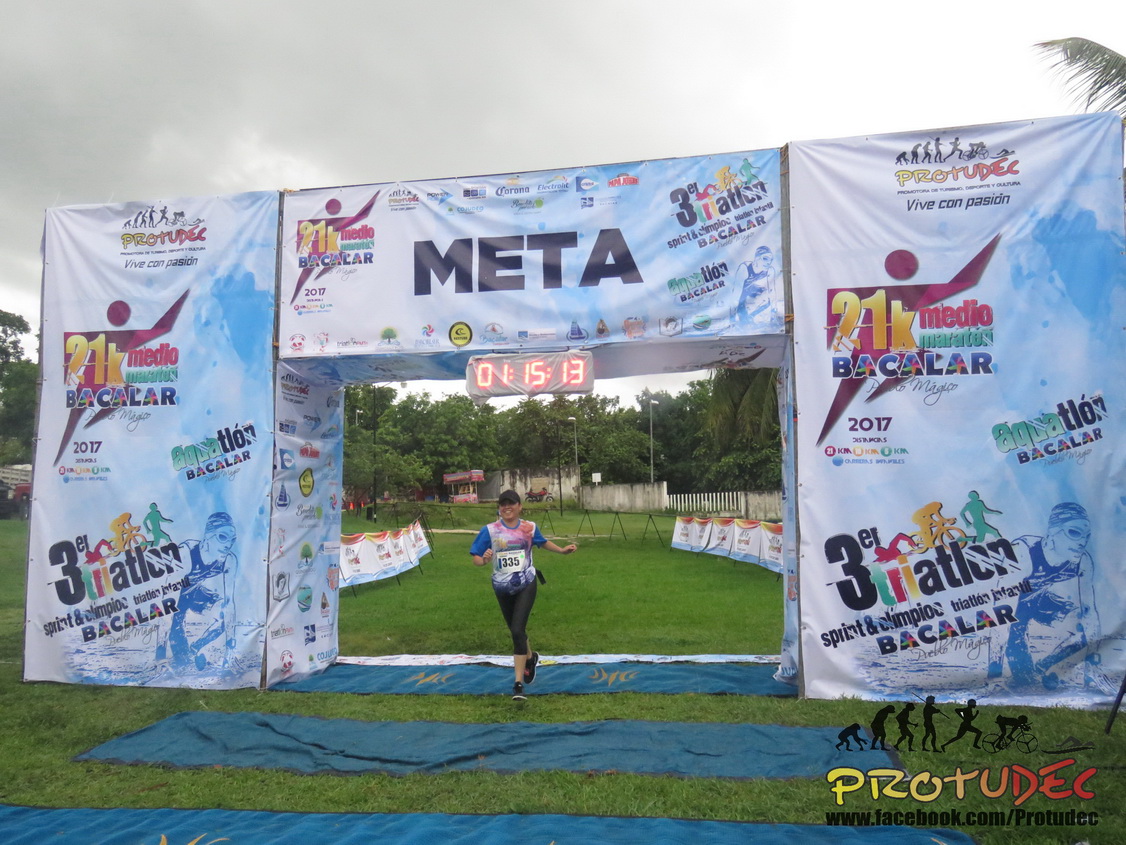The photograph captures the finish line of a triathlon event set on a green, grassy field with a backdrop of storm clouds and distant trees. In the foreground is a large, horizontally aligned, plastic structure resembling a garage door, adorned with various writings and colors. The top of the structure prominently displays "META" in capital, dark blue or black letters. Below, an illuminated timer shows "01:15:13." The wall is festooned with other inscriptions like "21K," "METEO," "Bacalar 2017," and "Aquathlon," indicating the nature of the event. A woman, identified by her colorful pink and blue short-sleeved top, black leggings, black sneakers, and black cap, is running through the center, smiling, and wearing a number around her waist, presumably, having just crossed the finish line. To the right of the structure, the lower corner bears the text "ProTrudec" in yellow and red, along with a Facebook link that reads "www.facebook.com/ProTrudec." A blue tarp lies on the grass, likely to cover mud or wet ground. The scene is indicative of both the celebration and the physical toll of the race, encapsulated by the lone runner against a moody, weathered backdrop.